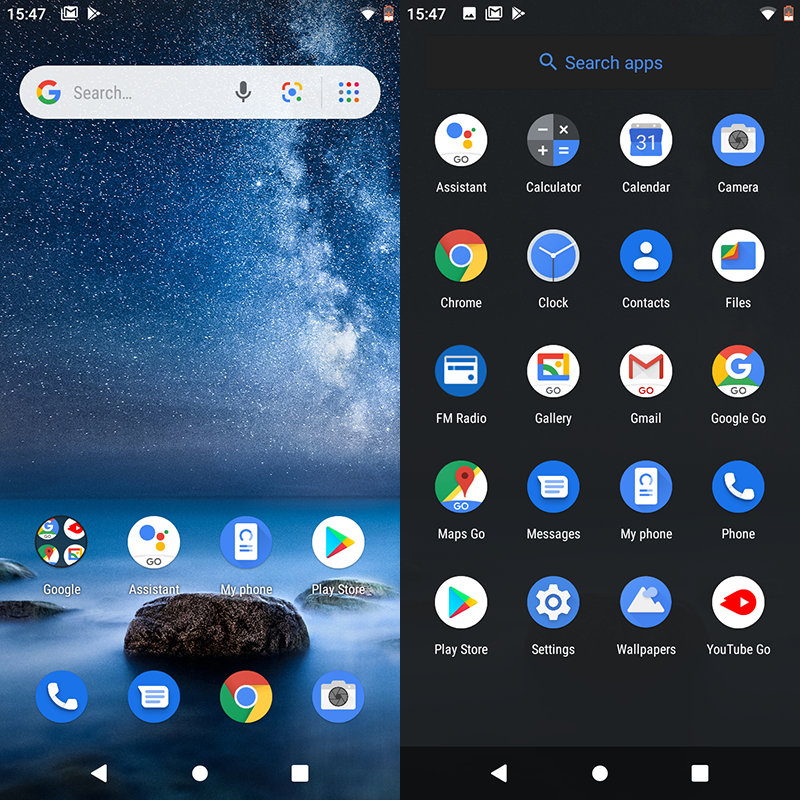The image depicts a split-screen display of a website. The right side of the screen is completely black and includes various search applications. The left side features a stunning screensaver reminiscent of a serene nighttime scene with water, rocks, and a sparkling sky with fading hues of white. Displayed prominently in the top left corner is the time, reading "15:47". 

The upper section of the screen is populated with a series of icons, including a notable red icon situated in the upper right corner, resembling a box with red above it. A Google search bar is visible, showcasing the recognizable "G" logo and a microphone icon.

Beneath the search bar, there's a Google box adorned with a myriad of colorful dots in shades of red, purple, and green. Additional elements at the bottom include icons labeled as Google, the Assistant, My Phone, Play Store, an image of a phone, a blue icon with a pad of paper, Chrome, a Google sign, a photograph, and a camera.

On the black right side, the top section mirrors the icons found on the left side. Underneath a search tab, the section lists various applications such as Assistant, Calculator, Calendar, Camera, Chrome, Clock, Contacts, Files, FM Radio, Gallery, Gmail, Google Go, Maps Go, Messages, My Phone, Phone, Play Store, Settings, Wallpapers, and YouTube Go.